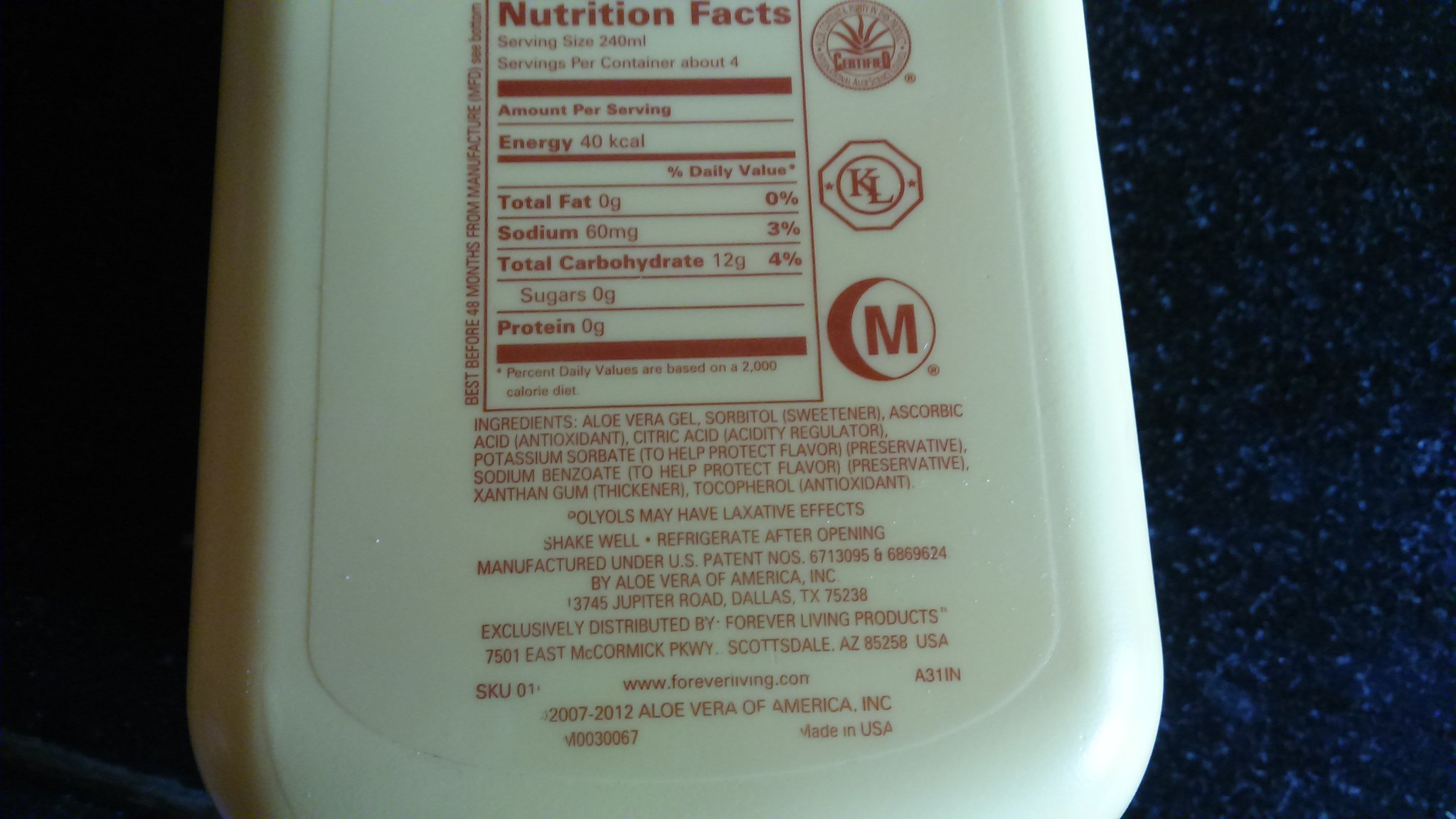This is a close-up photograph of a Nutrition Facts label on a white, flat container, possibly a plastic bottle. The label, printed in brown ink, details serving size as 240ml with about 4 servings per container. It lists the following nutritional information per serving: Energy - 40 kcal, Total Fat - 0g (0% DV), Sodium - 60mg (3% DV), Total Carbohydrates - 12g (4% DV), Sugars - 0g, Protein - 0g. The label also features three certification icons: one looks like a circle with a crescent moon and an "M" in maroon, another is a hexagonal symbol with "KL" and two dots within a circle, and the third is a certified circle symbol. Above the Nutrition Facts, there is barely distinguishable text along with an unidentifiable plant icon inside a circle. To the left of the Nutrition Facts, it states, "Best before 48 months from manufacture. Info, see bottom." Below the nutritional information are the ingredient details: aloe vera gel, sorbitol (sweetener), ascorbic acid (antioxidant), citric acid (acidity regulator), potassium sorbate, sodium benzoate (both preservatives), xanthan gum (thickener), and tocopherol (antioxidant). It also includes caution about a potential laxative effect, instructions to shake well and refrigerate after opening, and manufacturer information. The product is made under US patents by Aloe Vera of America Incorporated and distributed by Forever Living Products. Contact details include addresses in Dallas, Texas, and Scottsdale, Arizona, along with a website (www.foreverliving.com), and various identification numbers indicating its production and distribution. The container rests on a dark marble countertop with dark blue splotches.